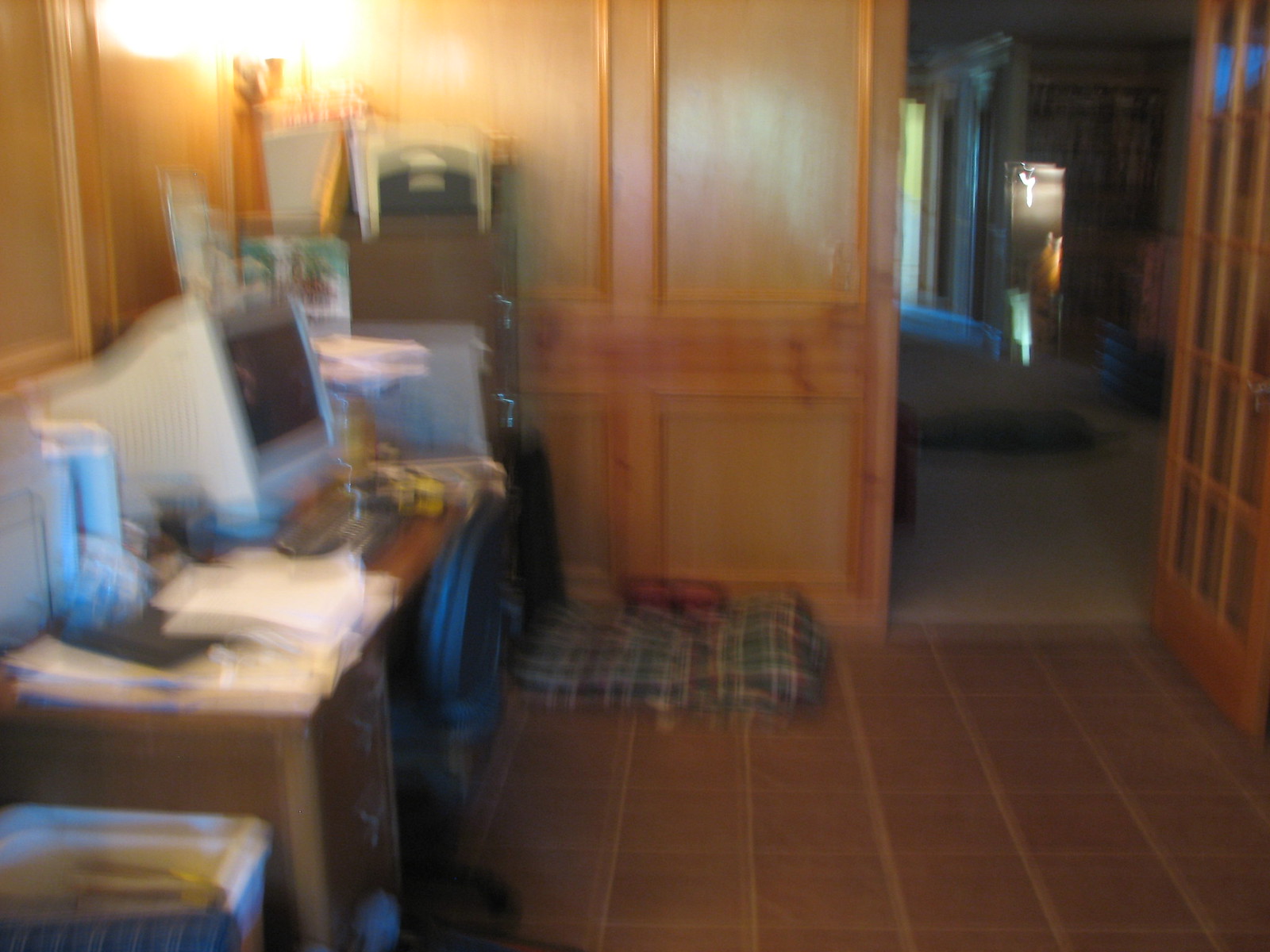In this heavily blurred photo, a doorway with an open brown-framed door is visible. The door features small rectangular windows outlined with wood. While the interior of the room beyond the doorway is unclear due to the blur, the doorway area reveals a carpeted floor. Preceding this is a room with brown square tiles. In this foreground room, a green and red checkered dog bed is positioned on the floor. An office setup occupies the left wall, consisting of a wooden desk with an old, bulky white computer monitor and an office chair pulled up to it. The desk is cluttered with stacks of papers, and beside the desk on the right side of the photo (left of the computer) is a file cabinet. Additionally, stacks of bins are placed against the wall, perhaps containing various items. A drawing is pinned up on the file cabinet, adding a touch of personal decor to the cluttered office space.